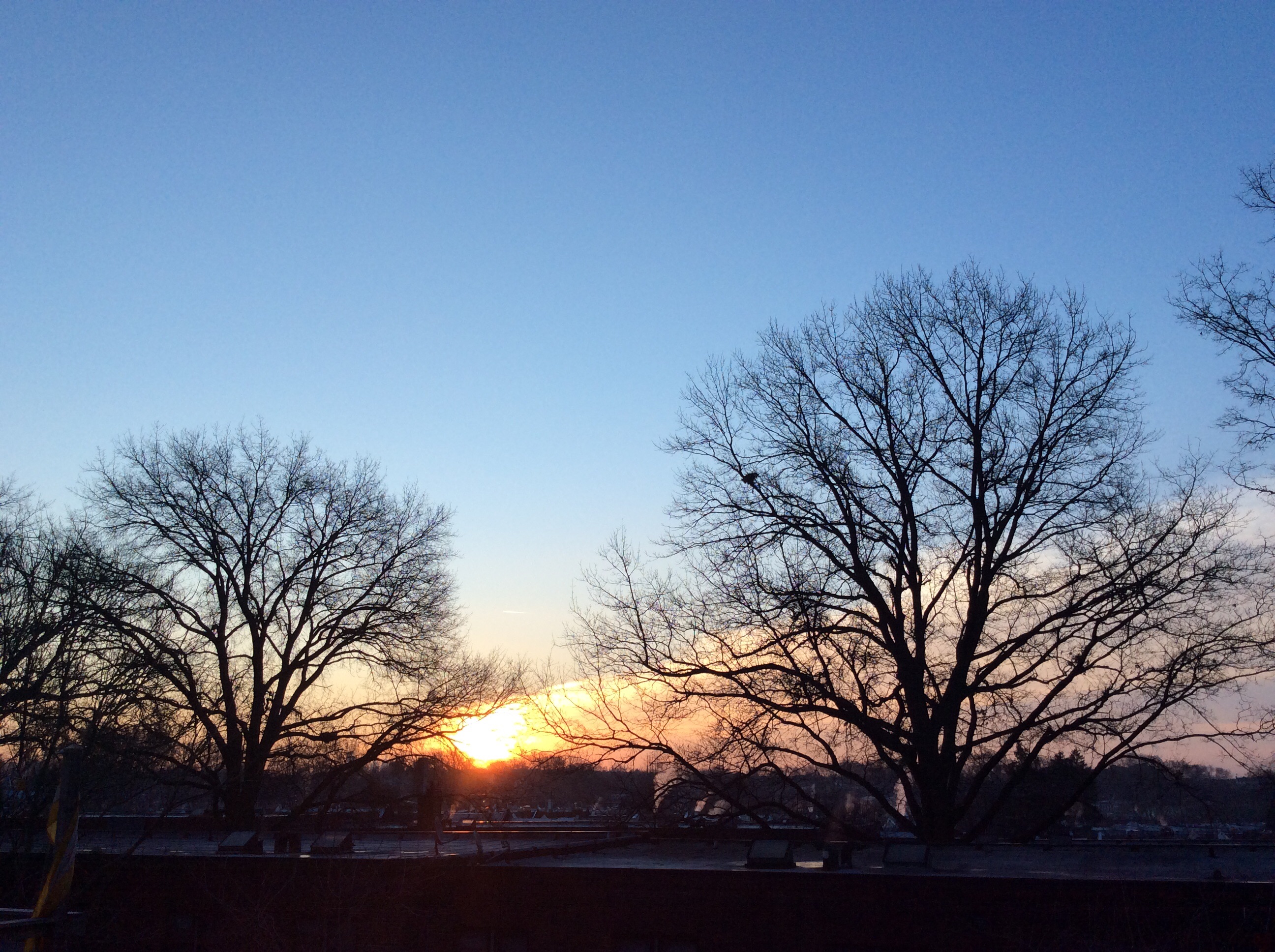The image captures a serene evening scene at twilight, likely in a park. The sun, a yellow orb, is setting just above the horizon in the lower-middle part of the square frame, lending a gentle, warm glow to the scene. The sky, occupying the majority of the picture, transitions from a clear, slightly darker blue at the top to a soft orange near the horizon, where streaks of white clouds tinged with orange flank the sun. The horizon lies about one-third up the image, beneath which the landscape turns almost black, silhouetting the elements below. In the foreground, large, bare trees with sprawling branches stand prominently, their stark outlines adding to the tranquil yet somewhat stark atmosphere. The bottoms of these trees merge into the darkened ground, suggesting the onset of night. The possible presence of rooftops in the distance hints at a nearby urban setting, though the overarching focus remains on the sky's beauty and the silhouetted trees, capturing the quiet transition from day to night.